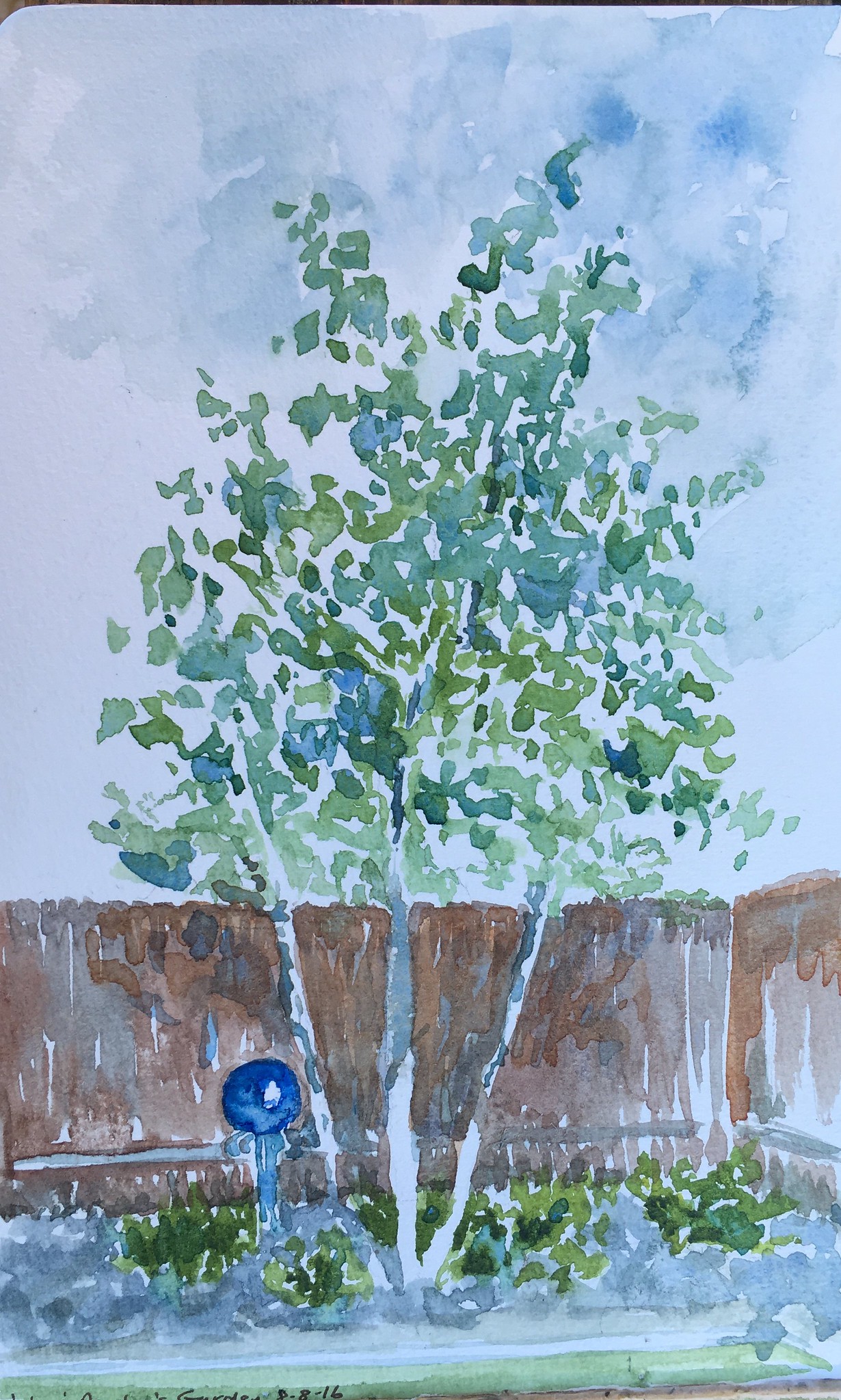This vertically oriented watercolor painting depicts a single, large, flowering tree with three trunks merging at the base. The tree's trunk is painted in shades of blue, with leaves rendered in green and blue hues, forming a vibrant canopy. At the base of the tree, a patch of green grass is dotted with blue leaf-like objects. There is a curious blue circular object near the base, mounted on what appears to be a gray pole. Behind the tree stands a brown wooden picket fence, complete with supportive crossbars inside. The background features a blue sky speckled with abstract cloud formations. The scene gives an impression of a peaceful garden or backyard setting, captured in the serene and soft textures of watercolor on an A4-sized canvas.